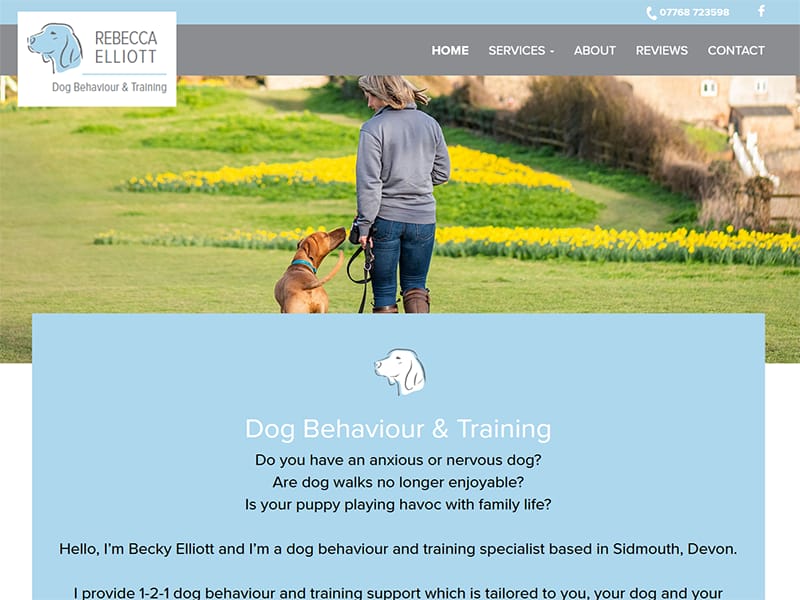The image is of the homepage of a dog training service website. At the top of the page, there is a light blue navigation bar featuring a white telephone icon followed by a contact number and the Facebook logo. Below this is a gray navigation bar with the following menu options in white, uppercase font aligned to the right: "Home," "Services" with a dropdown menu, "About," "Reviews," and "Contact." Overlapping these two top bars and the main image is a logo on the left, consisting of a cartoonish drawing of a dog's head in blue with a gray outline. Accompanying the logo, in gray, uppercase font, is the name "Rebecca Elliot," underlined by a blue line, followed by "Dog Behavior and Training" in gray, initial capital letters.

The main focal point of the page is a scenic image of a grassy area, possibly a park. In this setting, a woman clad in boots, jeans, and a gray long-sleeve shirt is walking a dog. The dog appears to be a brown-blonde Labrador, calmly walking beside her. The overall design of the website suggests a professional yet friendly dog training service.